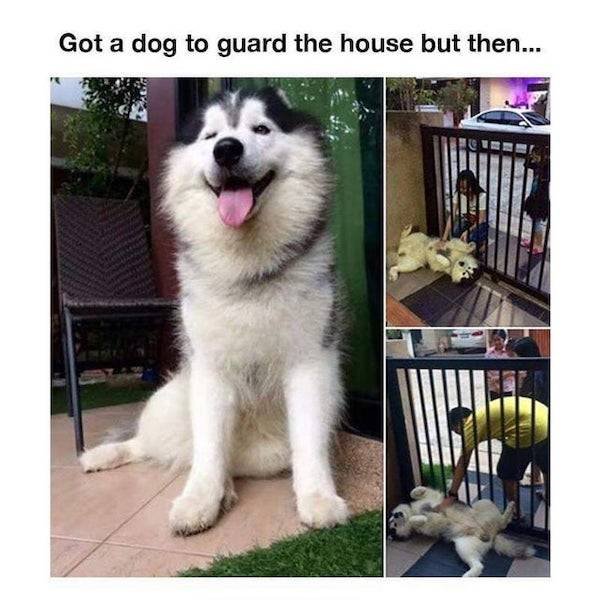A humorous and endearing photo collage featuring a large, happy-looking husky in three different panels. The main image on the left two-thirds shows the dog sitting contentedly with its tongue hanging out to the side, occupying most of the frame. The husky, with its black, white, and gray fur, is situated on a tile floor with a grassy area and a bench in the background. The two panels on the right capture the same husky in different scenes. In the top right image, the dog is lying on its back against a fence, enjoying belly rubs from a girl wearing a white t-shirt and blue pants, while another girl in a black dress with pink sandals stands nearby. A street scene with a car is visible in the background. The bottom right image shows the dog in a similar position, this time receiving belly rubs from a man dressed in a yellow shirt and black shorts. Both right images depict onlookers reaching through the fence to pet the friendly husky, contrasting humorously with the caption above the main panel that reads, "Got a dog to guard the house, but then..." This clever juxtaposition highlights the dog's affectionate nature, making it clear that this so-called guard dog is more interested in belly rubs than in guarding the house.